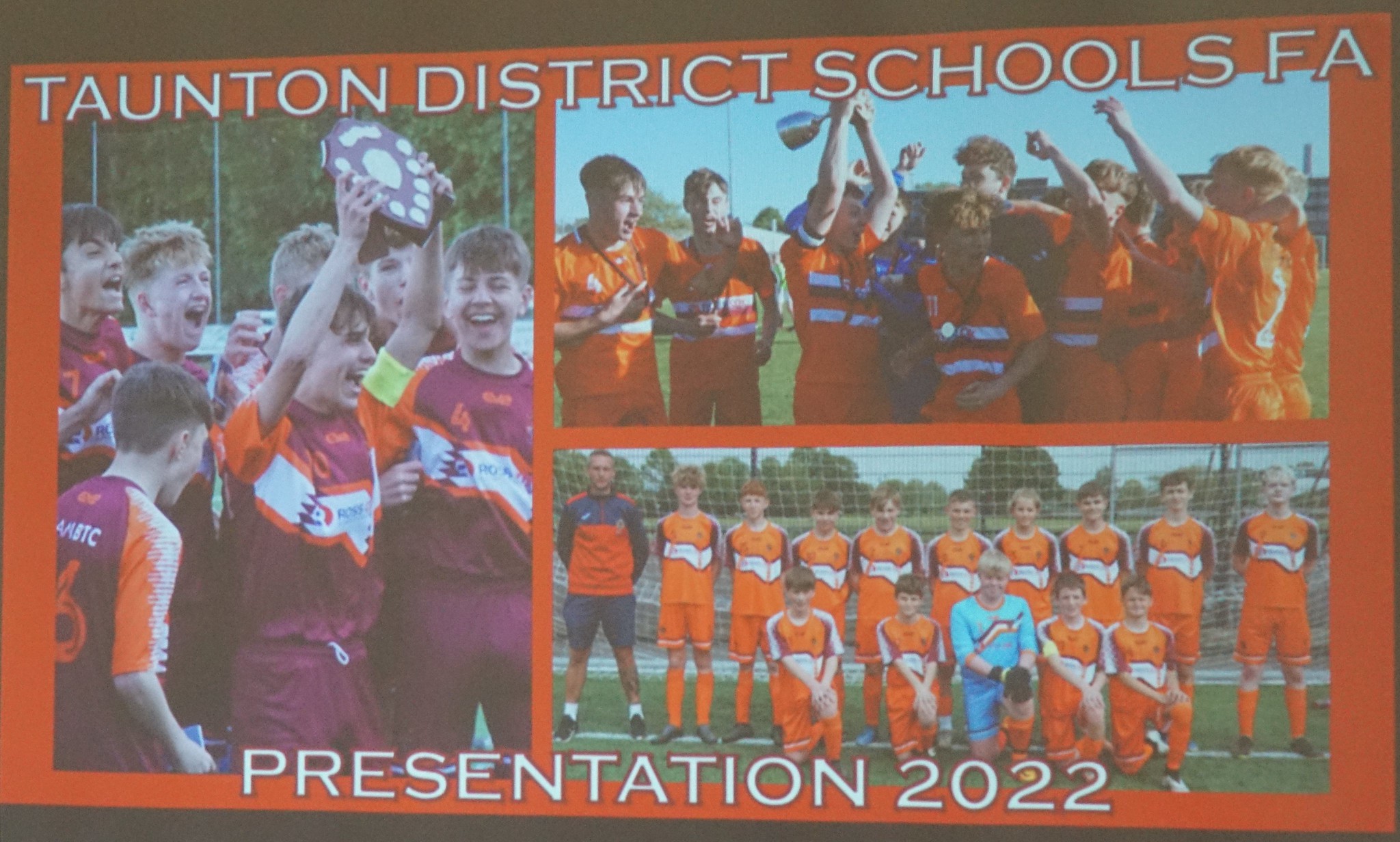The image is a collage of three distinct photographs showcasing championship celebrations by the Taunton District Schools' soccer teams, emphasized with "Taunton District Schools, F.A." at the top and "Presentation 2022" at the bottom. The left photograph is vertical and depicts a group of jubilant teenage boys holding up a plaque adorned with shields, clearly energized and exultant about their victory. The top right photograph is horizontal and shows another group of equally excited players on a sports field, hoisting a championship cup high into the air, their expressions filled with joy and triumph. The bottom right photograph, also horizontal, features a soccer team lined up in front of a goalie net, dressed in matching orange and maroon uniforms, standing with their hands behind their backs, projecting pride and unity. The images collectively capture the enthusiasm and accomplishments of the school’s athletic program.